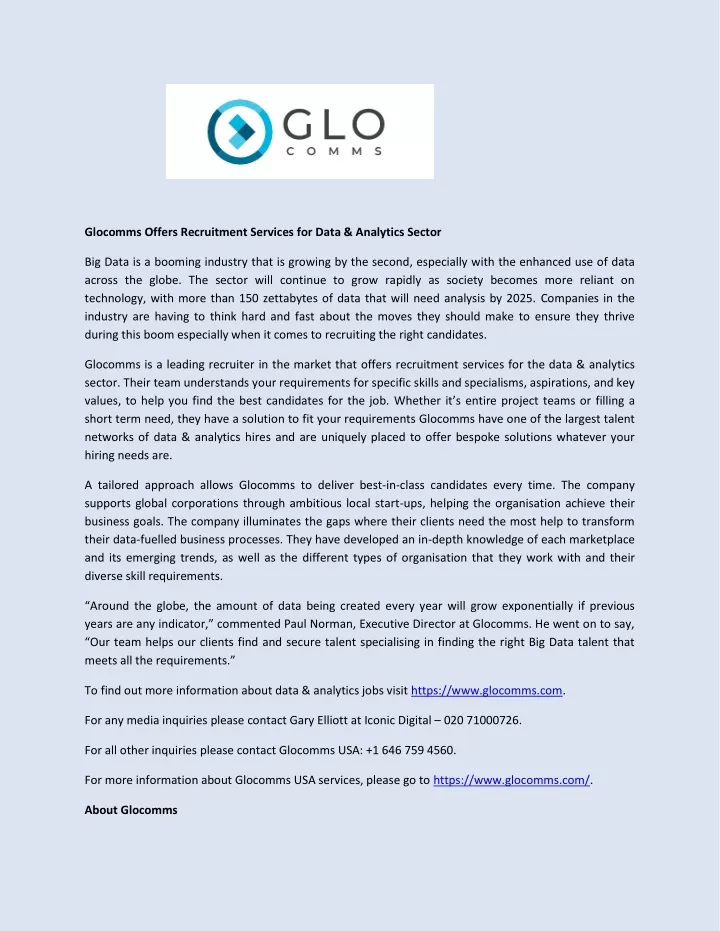In this image, we have a screenshot from a message on a website or app. At the top, there is the company logo for Glowcoms, which is designed in varying shades of teal. The logo features a circle with a right-pointing triangle that has one side missing. Glowcoms is spelled "G-L-O". The background of the image is light gray.

Beneath the logo, there is a text block describing the services offered by Glowcoms. The text reads: 

"Glowcoms offers recruitment services for the data and analytics sector. Big data is a booming industry that is expanding rapidly, particularly due to the increased global use of data. With more than 150 zettabytes of data expected to require analysis by 2025, companies must strategize carefully to thrive in this explosive growth period. Recruiting the right candidates is crucial.

Glowcoms is a leading recruiter for the data and analytics sector. Their team understands the specific skills, specialisms, aspirations, and key values needed to find the best candidates for the job, whether it's assembling entire project teams or meeting short-term needs. Glowcoms boasts one of the largest talent networks in data and analytics and is uniquely positioned to offer bespoke solutions tailored to your hiring needs. 

Their tailored approach ensures they deliver top-tier candidates every time. They support organizations ranging from global corporations to ambitious local startups, helping them achieve their business goals. Glowcoms identifies gaps where clients need the most support to transform their data-driven business processes. They possess in-depth knowledge of each marketplace, emerging trends, and the diverse skill requirements of their partners.

'The amount of data being created globally will grow exponentially if previous years are any indicator,' commented Paul Norman, Executive Director at Glowcoms. 'Our team specializes in finding and securing the right big data talent that meets all requirements.'

For more information, contact us."

This comprehensive caption accurately reflects the content and context of the original text, providing clear and detailed information about the services offered by Glowcoms.